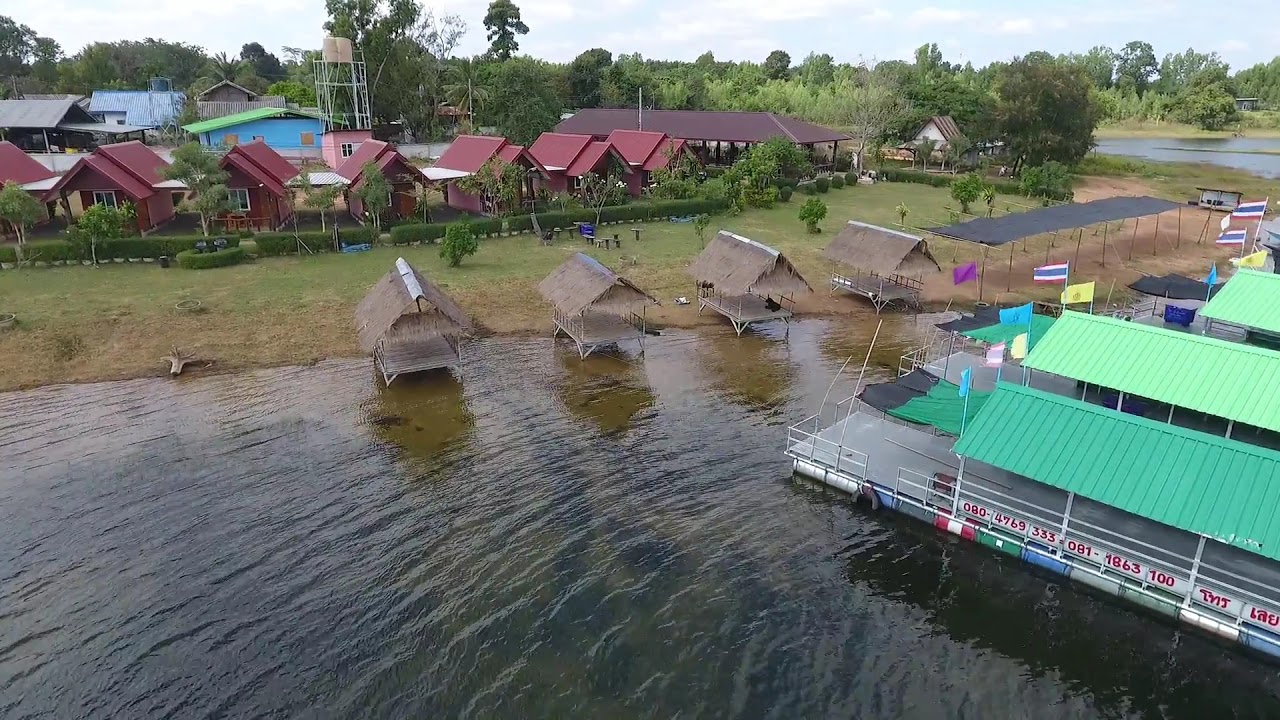This horizontal-rectangular image showcases a picturesque lakeside area bordered by water, which occupies roughly 45% of the frame. The water, a brownish hue suggestive of muddiness, laps against a shoreline that features boat docks suitable for speedboats or rowboats. Notable on the water are large pontoon boats with canopy coverings, appearing rentable for lake excursions.

To the right side of the image, a grassy area transitions to a row of buildings, predominantly residential, characterized by uniform roof colors and clean, geometric designs. In addition, there is a conspicuous blue building nestled among these houses.

In the middle section of the picture, a green-roofed structure seems to float on the water, accompanied by four straw and wood bungalows elevated above the surface. Beyond this, an array of charming red houses with red roofs and tiny decks are neatly arranged, adding a splash of color and charm. Vegetation, trees, and an old water tower populate the background, lending a lush, natural backdrop to the scene.